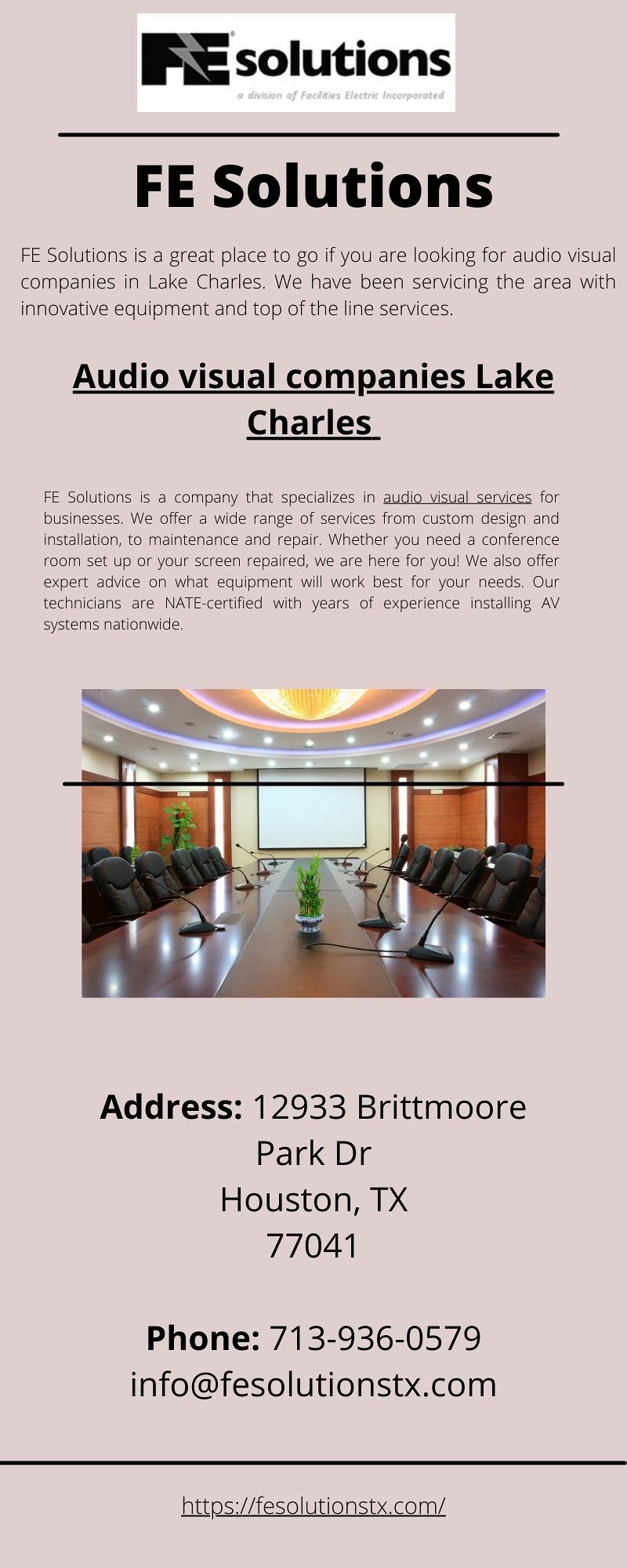The image showcases a detailed flyer for FE Solutions, a specialist in audiovisual services. The flyer features a muted pink background with the company name prominently displayed at the top: "FE Solutions." Described as an excellent resource for those seeking high-quality audiovisual services in Lake Charles, FE Solutions offers innovative equipment and top-of-the-line services. The flyer highlights their extensive expertise, including custom design, installation, maintenance, and repair of AV systems. The center of the image includes a photo of a modern conference room, complete with chairs, microphones, and a projector screen, underscoring the company's professional capabilities. The flyer further provides the company's contact information, including their address at 12933 Brittmoore Park Drive, Houston, Texas 77041, and their phone number, 713-936-0579. For more information, the flyer directs to their website at https://fesolutionsstx.com and offers additional contact via email at info@fesolutionstexas.com.